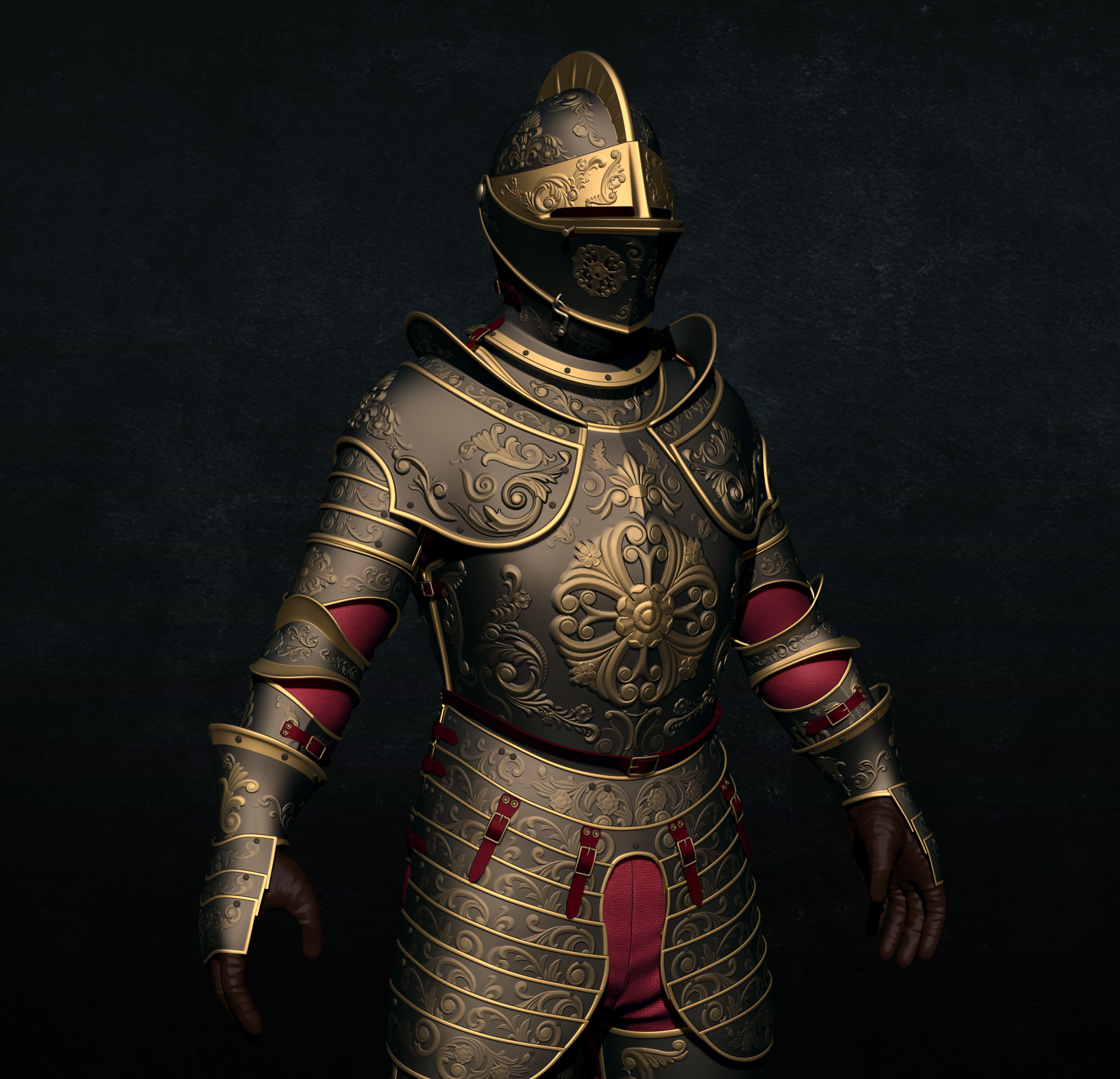The image showcases an intricately designed digital rendering of a knight in armor, possibly intended for a video game or concept art for a movie. Set against a predominantly black background with hints of gray tones and white speckles, the knight's armor features a striking dark brownish-gray surface, adorned with ornate gold highlights and floral leaf patterns.

The helmet is particularly notable, characterized by a black base with a gold ridge running across the top like a mohawk and a gold face shield, which has a slit where the eyes would be. The chest, arms, and pauldrons of the armor continue the theme with dark brown and gold accents, while the pauldrons stick up near the shoulders and have a fancy golden matte design at their center.

Peeking out from beneath the segmented skirt of the armor, which is outlined in gold, are red pants and red straps that run across the top portion of the skirt. The knight also sports a red belt around the waist, and their sleeves are red just above and below the elbows, where the armor features a double-flanged piece with a brass-like outline.

The gauntlets mimic the segmented design of the skirt, albeit on a smaller scale, and reveal brown leather gloves underneath. Overall, the intricate details and rich color contrasts make the knight's uniform a visually compelling digital artwork.